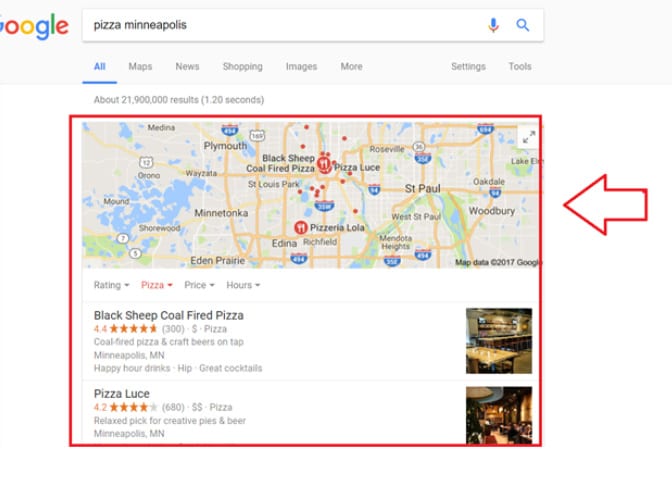The image displays a Google search page with the query "pizza Minneapolis" entered into the search bar. The Google logo in its iconic colors is visible at the top, along with the microphone icon. The blue search bar is prominently featured, followed by menu options such as "All", "Maps", "News", "Shopping", "Images", and "More" in gray text, except for "All" which is highlighted in blue and underlined. Below these options, it indicates there are about 21,900,000 results, found in 1.20 seconds.

Highlighted with a red box and an accompanying large red arrow, the image spotlights a section featuring Google Maps, showcasing locations of pizza places in Minneapolis. Red markers with knife and fork icons denote the locations. Visible areas on the map include Minnetonka, Plymouth, and Eden Prairie, displaying at least three pizza place markers.

Below the map, filters for "Rating," "Pizza," "Price," and "Hours" are shown in gray, except "Pizza," which is in red. The first search result is "Black Sheep Coal Fired Pizza" with a rating of 4.4 indicated by orange stars and "300 reviews." It includes a single dollar sign, specifying it offers "coal-fired pizza and crafty beers on tap." The location details mention happy hour drinks and a hip atmosphere with great cocktails in Minneapolis.

The second highlighted result is "Pizza Lucé," rated 4.2 with orange stars and "680 reviews." It is marked with two dollar signs and described as a "relaxed pick for creative pies and beer" located in Minneapolis. A small interior image of the restaurant accompanies this description.